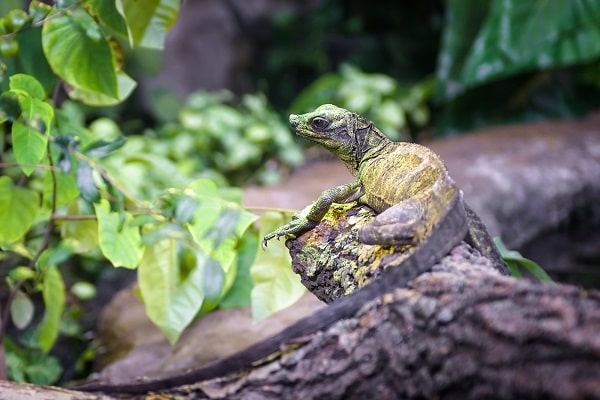The image depicts a lizard, possibly a gecko or iguana, perched on a brown tree branch in an outdoor, wildlife setting that almost resembles a terrarium. The lizard has a green head and a yellow back adorned with light brown spikes. Its long, dark grey tail extends to about three times the length of its body. The creature is looking to the left, showcasing its alert, forward-facing black eye. The back of the lizard features a prominent lump, while its green legs blend seamlessly with the branch, their nails just visible. The background consists of a vibrant green foliage with leaves that vary in shades of green, some tinged with yellow due to sunlight. On the left side, the leaves are primarily dark green and slightly yellowish-green, while the right side features the largest, darkest green leaf. The lizard almost blends in with its surroundings, accentuated by the close-up perspective of the photograph.